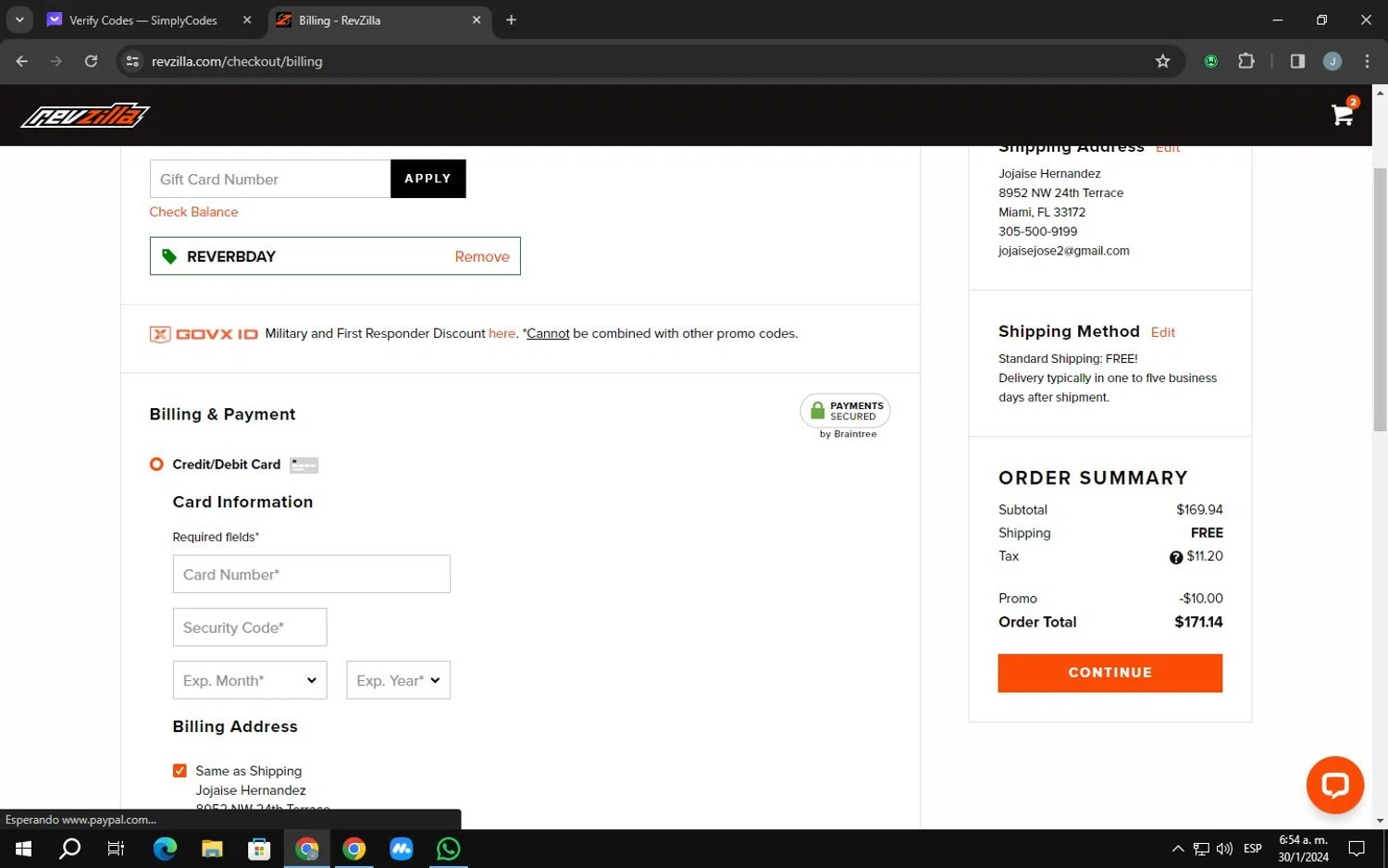The screenshot displays the "Billing" page on RevZilla's website, as indicated by the active browser tab labeled "Billing RevZilla." The URL in the search bar reads "revzilla.com/checkout/billing." Below the search bar, the RevZilla logo spans the screen, set against a black background. To its right, a shopping cart icon shows a notification of two items.

The page prominently features a gift card input field, accompanied by a rectangular "Apply" button and a "Check Balance" link. Below this, an input field contains the promo code "REVERBDAY" in all caps. To its left is a green sticker or price tag marker, and to the right is a clickable "REMOVE" link to clear this field. Beneath this is an area promoting a "GOVXID, Military and First Responder Discount," with the "Here" link clickable. A disclaimer states, "CANNOT BE COMBINED WITH OTHER PROMO CODES," with "CANNOT" underlined and marked by an asterisk.

Further down, the page displays sections for entering billing and payment details, including options for credit or debit cards with fields for card number, security code, and expiration date. The billing address section appears below these fields, and to the right is the shipping address section. The page also includes sections for the shipping method, an order summary, and a rectangular "CONTINUE" button for proceeding with the checkout process.